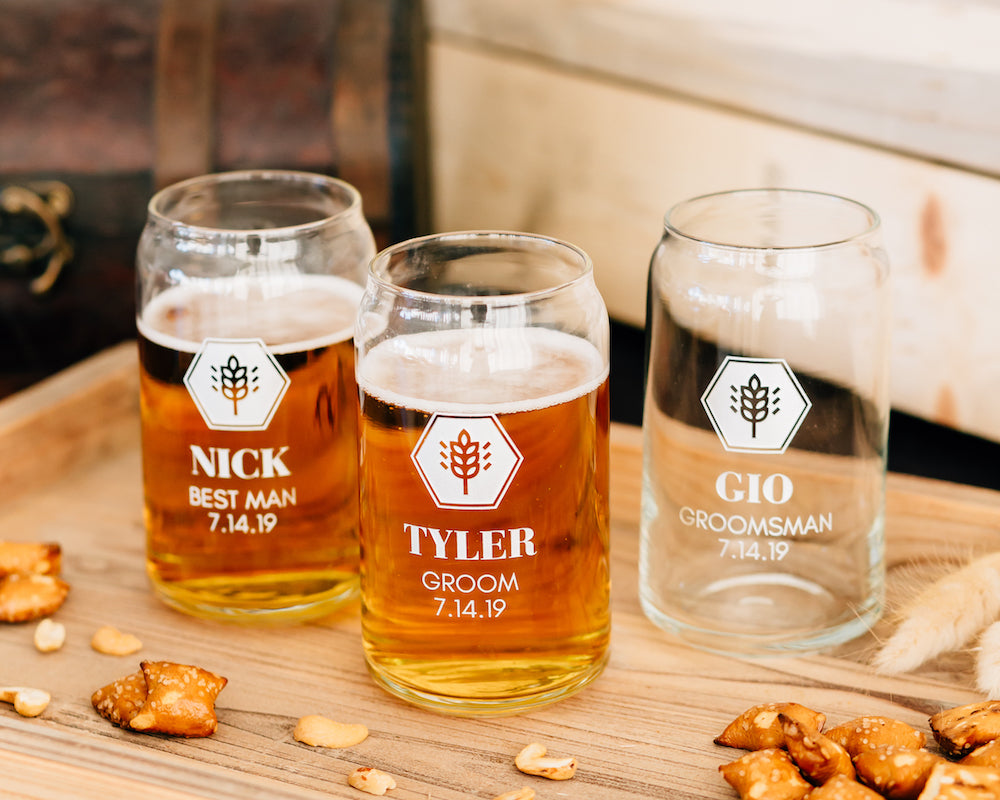The image depicts three personalized beer glasses, likely intended as groomsmen gifts for a wedding, arranged in a landscape orientation. Each clear glass has a slightly narrow neck at the top and features a white hexagon emblem with a tiny leaf icon. Below the emblem, inscriptions in white text specify the name, role, and wedding date: "Nick, Best Man, 7-14-19" on the left, "Tyler, Groom, 7-14-19" in the middle, and "Gio, Groomsman, 7-14-19" on the right. The left and middle glasses contain amber-colored beer with foam, while the right glass is empty.

The glasses rest on a light wooden tray scattered with square pretzel bits and half peanuts, atop a light-colored, finished wooden table. In the blurred background, a wooden dresser is visible on the right, and a wooden chest on the left. Additionally, a cattail plant (not the animal, but the plant) is seen towards the right side of the image, contributing to the overall rustic setting.